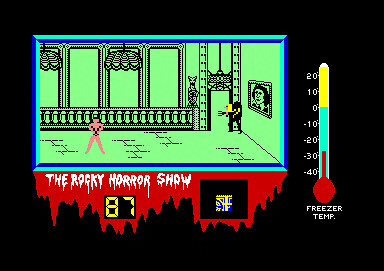This detailed and cleaned-up caption for the image can be:

---

**Caption:**

This image captures a screenshot from an older, pixelated video game heavily styled in green hues, depicting a castle hallway with distinct retro graphics. The scene features two characters: one is pink, and the other appears hunched with long yellow hair, seemingly holding a pitchfork. The hallway is decorated with several chandeliers hanging from the ceiling. On the right wall, a framed portrait of a character resembling Dr. Frankenfurter from the Rocky Horror Show is prominently displayed. The central green area of the game is enclosed by a blue frame, occupying a small portion of the overall black screen. Below this green game area, stylized blood drips down to form the title "The Rocky Horror Show" in white, dripping text. Additional interface elements include a yellow "87" inside a square, and another black square displaying an indistinguishable item. To the right, there's an indicator labeled "Freezer Temp" with a thermometer showing approximately -28 degrees.